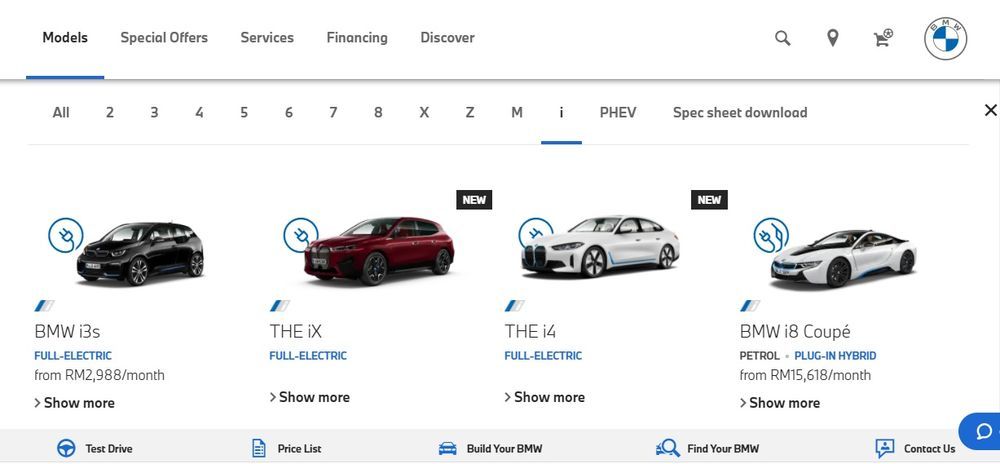This is an image of a detailed specification sheet on a BMW car website. At the very top left, the navigation menu starts with several clickable tabs: "Models" highlighted in black with a blue underline, followed by "Special Offers," "Services," "Financing," and "Discover" all in gray. Below this menu is a gray dividing line, under which a secondary navigation bar is displayed with the options: "All," "2," "3," "4," "5," "6," "7," "8," "X," "Z," "M," "i," and "PHEV" in capital letters. To the right, there is a "Spec Sheet Download" option, with a blue underline beneath the "i."

Below this, four car images are presented with corresponding details:

1. **BMW i3s (Full Electric)**:
   - Image: Small black car
   - Emblem: Plug-in emblem on the left
   - Price: From RM2,988 per month
   - Action: "Show More" with a right-hand arrow

2. **BMW iX (Full Electric)**:
   - Image: Red car
   - Emblem: Plug-in emblem on the left
   - Action: "Show More" with a right-hand arrow

3. **BMW i4 (Full Electric)**:
   - Image: [Car image not specified; assumed similar presentation]
   - Emblem: Plug-in emblem on the left
   - Action: "Show More" with a right-hand arrow

4. **BMW i8 Coupe (Petrol Plug-in Hybrid)**:
   - Image: [Car image not specified; assumed similar presentation]
   - Emblem: Plug-in and petrol emblems on the left
   - Price: From RM15,618 per month
   - Action: "Show More" with a right-hand arrow

At the very bottom of the page, there are five additional clickable tabs: "Test Drive," "Price List," "Build Your BMW," "Find Your BMW," and "Contact Us."